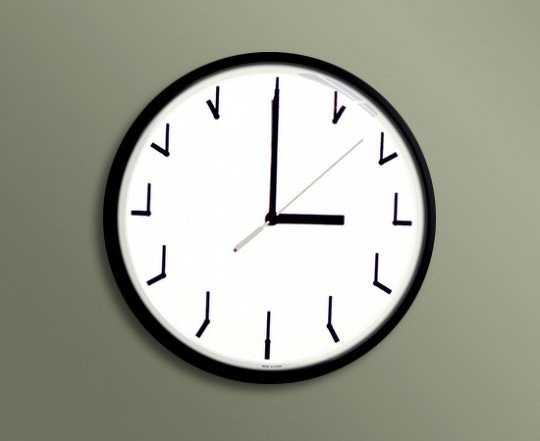This digital artwork features a creatively designed clock set against a light beige background. The clock itself is outlined in black, with a stark white face. Instead of the traditional numbers, each hour is represented by a unique illustration depicting what a clock would look like at that specific time. At the present moment, the clock displays 3 o'clock: the minute hand points straight up to 12, while the hour hand extends to the right, towards the position of the 3. Uniquely, at the 3 o'clock position, the illustration resembles a right triangle. Additionally, the second hand lies between where the 1 and 2 would traditionally be found on a standard clock, adding a dynamic element to this imaginative creation.